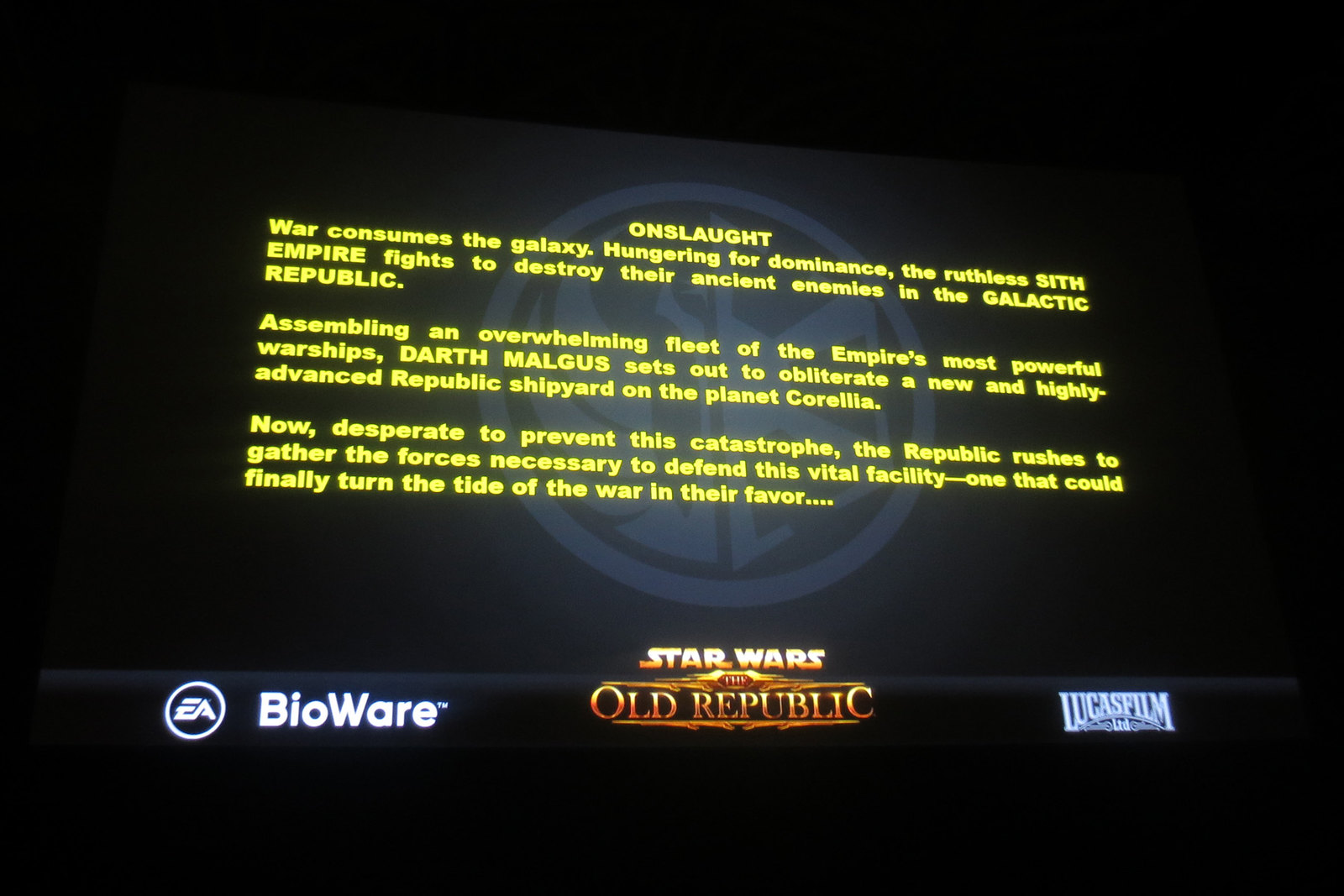The image is a detailed screenshot from a video game, featuring a predominantly black background with a central gray circle that contains an indistinct emblem. In bright yellow text at the top, it reads "Onslaught." Following this, a descriptive narrative is showcased: "War consumes the galaxy, hungering for dominance. The ruthless Sith Empire fights to destroy their ancient enemies in the Galactic Republic. Assembling an overwhelming fleet of the Empire's most powerful warships, Darth Malgus sets out to obliterate a new and highly advanced Republic shipyard on the planet Corellia. Now desperate to prevent this catastrophe, the Republic rushes to gather the forces necessary to defend this vital facility, one that could finally turn the tide of the war in their favor." At the bottom center, in a gold font, it reads "Star Wars: The Old Republic." The bottom left features the EA logo within a white circle, adjacent to the BioWare logo, while the bottom right displays the Lucasfilm LTD logo.